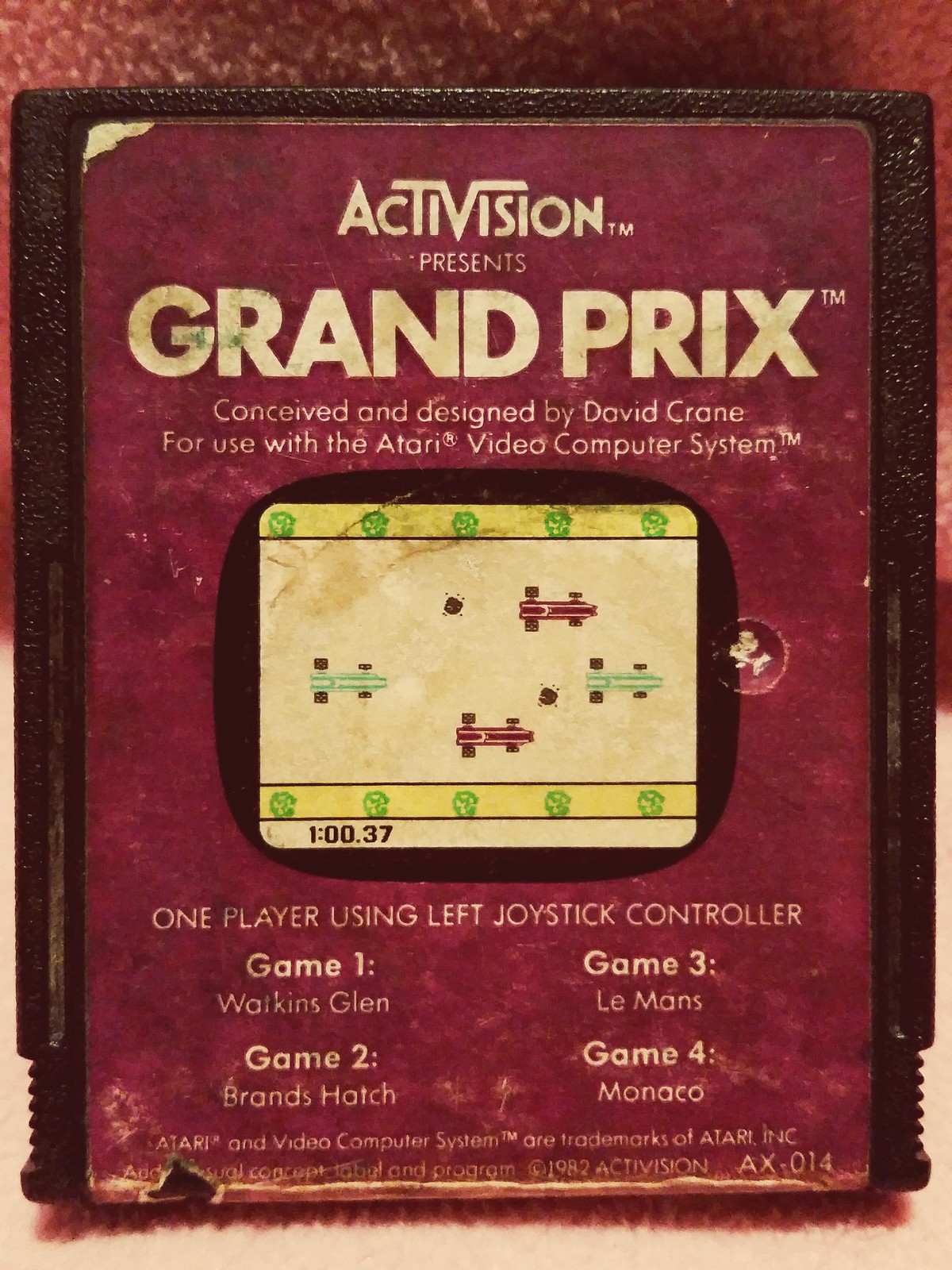This image is a detailed photograph of an old Atari video game cartridge for the game "Grand Prix," developed by Activision TM. The cartridge has a square, slightly rectangular shape with a black, textured finish around its borders. Dominating the center is a paper label in burgundy, slightly worn at the top left corner, revealing a tan color beneath. 

The label features white text, including the title "Activision TM presents Grand Prix TM conceived and designed by David Crane for use with the Atari video computer system." Additionally, it notes that the game is for one player using the left joystick controller and provides information about the four different racing tracks: Game one - Watkins Glen, Game two - Brands Hatch, Game three - Le Mans, and Game four - Monaco.

A graphic in the center of the label depicts a scene from the game, showing cars on the racetrack. There are two red cars and two green cars with black tires racing between two yellow borders with green plants on the top and bottom. The bottom left corner of the graphic includes some in-game time information. The cartridge is resting on a piece of paper with some red visible, adding to the vintage appeal of the photograph.